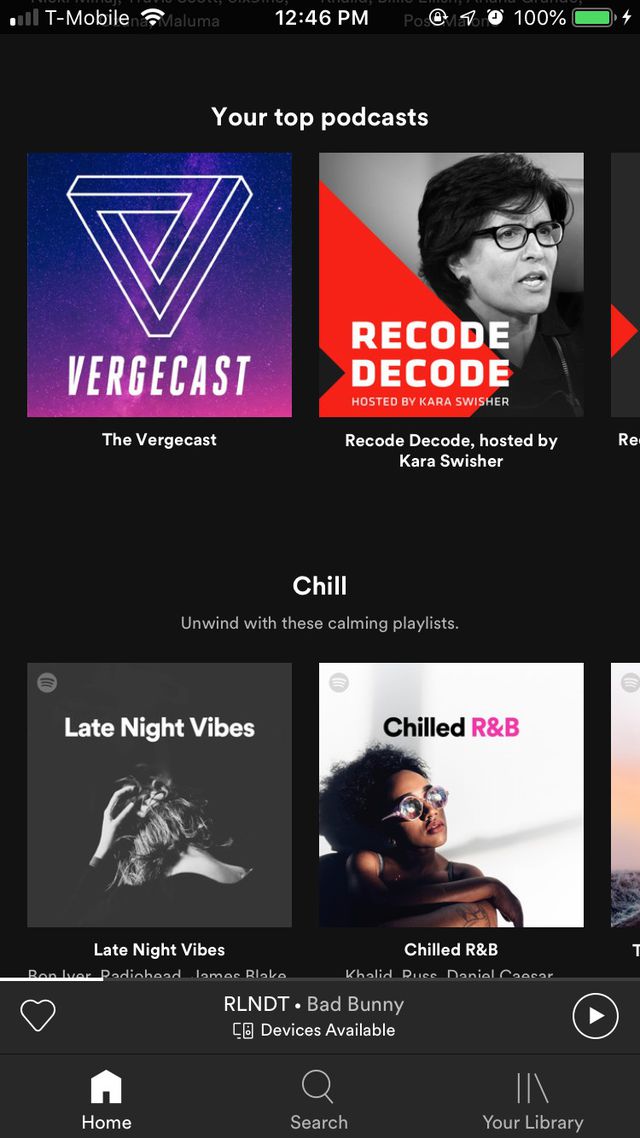A detailed mobile screenshot of a podcast website, viewed in dark mode. At the very top, the status bar displays network information with "T-Mobile" on the left and full signal bars. The time, centered at the top, reads 12:46 PM. To the right, battery status indicators show a full 100% charge with a green battery icon, a lightning bolt symbol indicating charging, and other standard icons.

The main content below features a black background. Prominently displayed is the title "Your Top Podcasts" with two podcast options visible. The first podcast is "Vergecast," represented by a logo resembling an upside-down triangle accompanied by the title "Vergecast" and a subtitle "The Vergecast." The second podcast, "Recode Decode," is hosted by Kara Swisher and has a black-and-white image of Swisher with short dark hair and glasses, mouth open as if speaking.

Below, the section titled "Chill" invites viewers to "Unwind with these calming playlists." Again, two options are presented. The first, "Late Night Vibes," has a hard-to-decipher black-and-white image of a woman seen from behind, her head in her hands. The second, "Chilled R&B," features a colored photograph of an African American woman, leaning against a wall. Only her upper body is visible; her arms are crossed, and she wears sunglasses, gazing slightly upwards. Each playlist title is clearly labeled below the images.